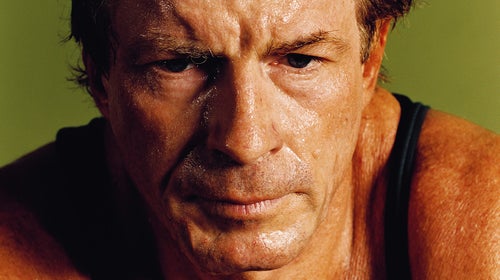This image features an up-close, detailed photograph of a white man in his mid-50s to early 60s, occupying most of the frame. His leathery, tanned skin—likely from extensive sun exposure—glistens with sweat that shines on his brow, nose, and mouth. He has brown hair, brown eyebrows, and dark brown eyes that look pensive or upset. His furrowed brow and deep nasolabial folds accentuate his worried expression as he gazes downward to the right, away from the camera. Stubble is visible above his lip and on his chin, further highlighting his age. He is wearing a black tank top, with muscular shoulders suggesting physical activity. The background is a nondescript olive green, making his expressive, sweaty face the focal point of the image.